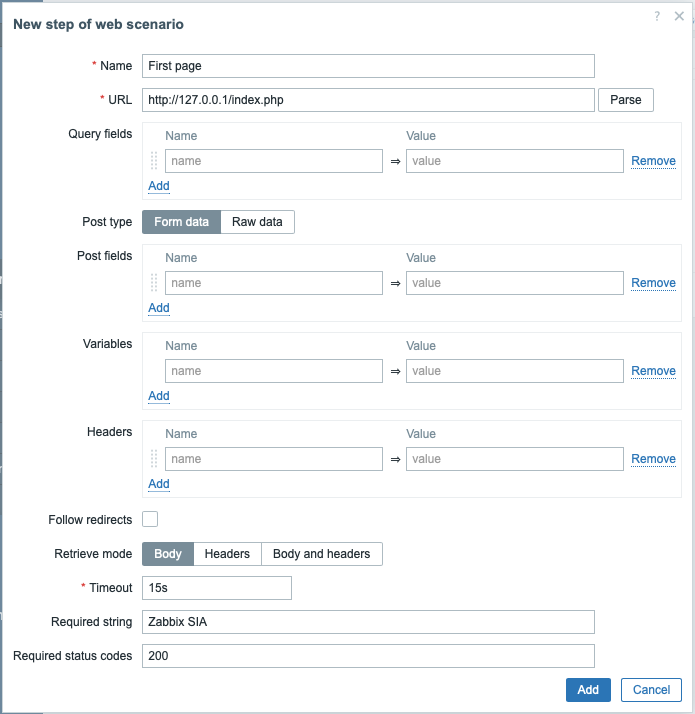**Descriptive Caption:**

A screenshot showcases the web scenario settings interface for Zabbix. The main elements include a form with multiple sections and fields. The URL field at the top reads "http://localhost/zabbix/index.php," adjacent to a "Parse" button. Below, there's a section dedicated to query fields, with separate inputs labeled "Name" and "Value," each followed by "Add" and "Remove" options.

Further down, there's a choice menu labeled "Post Type," allowing the selection between "Form Data" and "Raw Data." Selected is "Form Data." Additionally, a "Post Field" section includes fields for "Name" and "Value," along with the "Add" and "Remove" options.

The "Variables" and "Headers" sections are configured similarly, each providing inputs for "Name" and "Value," alongside corresponding "Remove" and "Add" buttons.

A "Follow Redirect" option is enabled, indicated by a blue tick. The "Receive Mode" setting is evident with options for "Body," "Headers," and "Body and Headers," with "Body" being highlighted. The "Timeout" field is set to 15 seconds.

Two crucial conditions are listed at the bottom: "Required String: ZABBIX SIA" and "Required Status Codes: 200." Finally, the options "Update" and "Cancel" are available at the bottom.

The interface features a color scheme primarily consisting of teal, shades of blue-gray, black, and white, all framed within a gray outline on a white background.